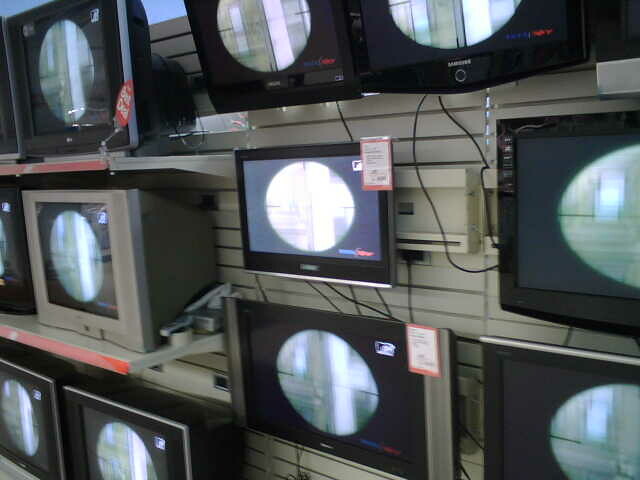This color photograph depicts a store display wall showcasing an array of dated televisions, varying from CRT models to early flat screens. Arranged in three distinct sections—left, middle, and right—the display features a total of 12 screens, each with a circular image in the center, resembling a viewfinder, possibly connected to cameras. 

On the left side, the TVs are organized in three rows: the top row includes a small black monitor with a box behind it, the middle row has a gray screen reminiscent of an old computer monitor, and the bottom row houses two black screens. 

In the central section, the middle screen is a modern flat screen mounted directly to the wall, flanked by two black screens above and a gray-bordered screen below, also attached directly to the wall. 

The right section follows a similar pattern with black TVs arranged in rows. The entire setup features attached black wires and blurred labels, including some from brands like Samsung, indicating this is likely a storefront. The background of the display wall is gray, enhancing the organized but somewhat dated appearance of the television array.